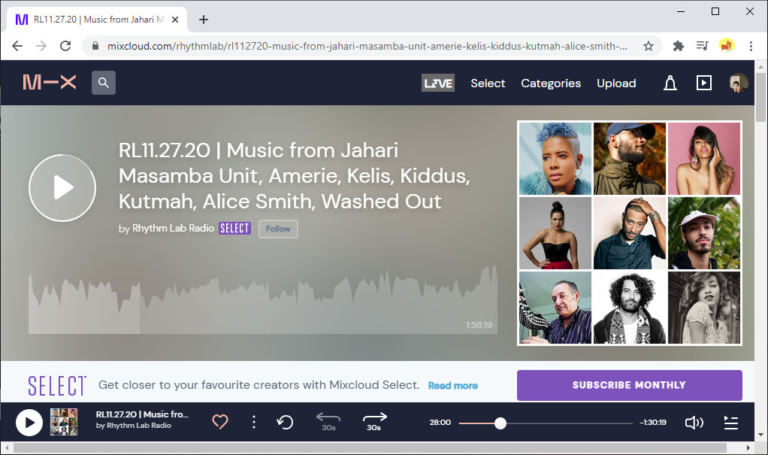**Caption:**

This image encapsulates a vivid snapshot of the Mixcloud interface featuring a radio show titled "RL112720 - Music from Jahari." The central section of the screen highlights various interactive elements such as a gray rectangle displaying a minus sign, square, and an X, alongside left and right arrows. Below this, a textual banner reads "mixcloud.com/rhythm_lab/RL112720 - Music from Jahari, Masamba, Union, Marion, Kelly, Kidiz, Kutma, Alice, Smith..." providing details on the featured artists.

Prominently, a black bar bearing the letters "M", a sideways "I", and an "X" is visible above a gray square with a magnifying glass icon, indicating the search functionality. The right side of the image includes additional navigation elements labeled "Live," "Select Category," "Upload," and a bell icon for notifications.

Intense visual activity populates the middle section, which details "RL112720" with references to artists Jahari, Masamba, Union, Marion, Kids, Kidiz, Kutma, and Alice Smith. Also mentioned is "Five Rhythm Lab Radio" and an invitation to "Select File."

Below this, there are visual thumbnails of various individuals: one with blue hair and a blue cap, another with long hair and a bra, a person with yellow hair, someone grabbing their head, someone taking a selfie, and another individual with a statue.

A call to action invites viewers to "Select, get closer to favorite creation," and explore "Mixcloud Select" with options to "Read More" or "Subscribe Monthly." The current playtime of the audio is at 28 minutes with an hour and 30 minutes remaining.

Added decorative icons such as stars, puzzles, dash marks, and music notes adorn the page, contributing to the vibrant, eclectic feel of the Mixcloud interface.